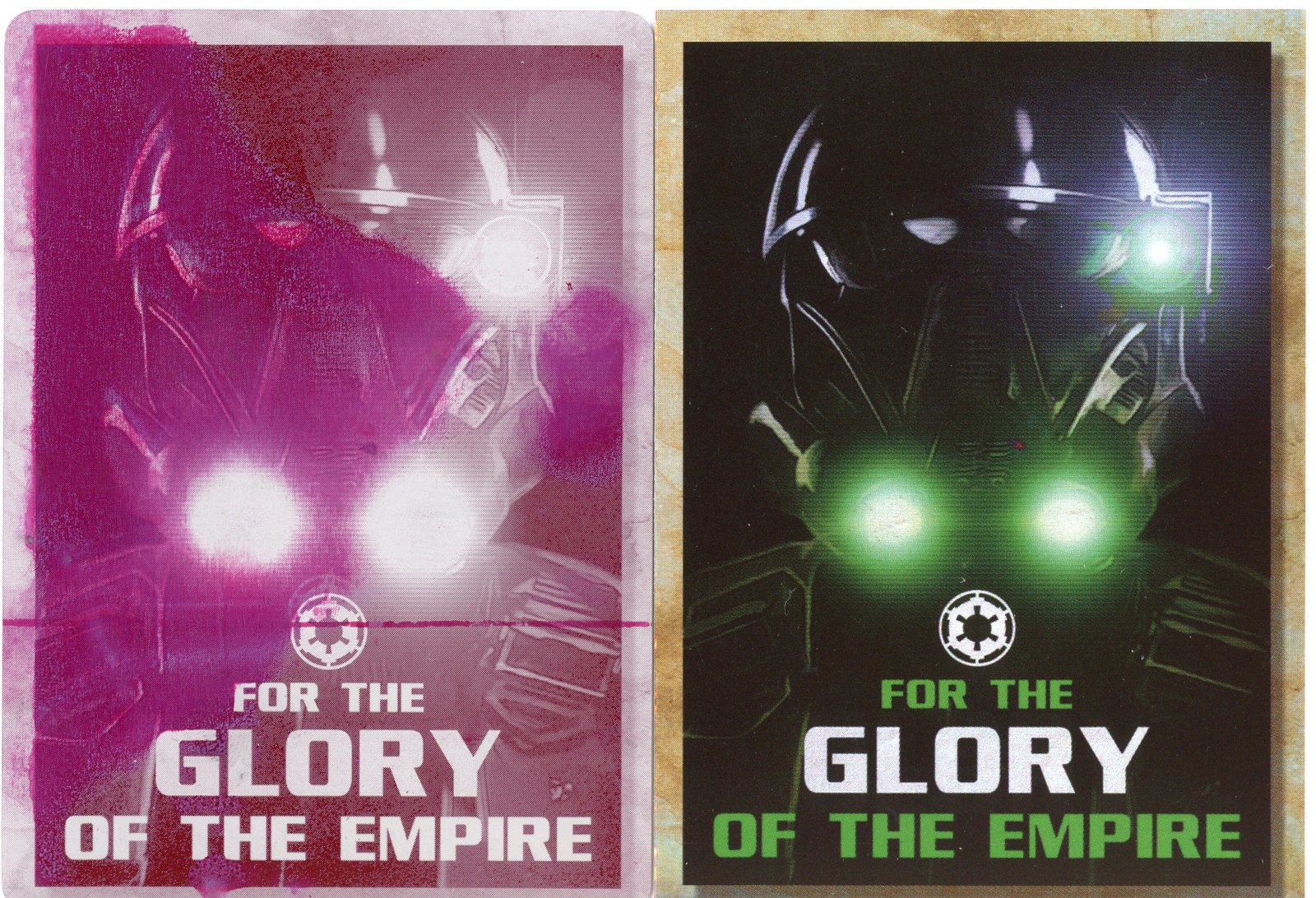This image showcases two visually striking, poster-like representations of a mechanized character that closely resembles a Black Stormtrooper from Star Wars. Both images feature the same centered figure adorned in sleek black armor with a stylized helmet. In the poster on the right, the character is highlighted by green neon lights emanating from the sides of the helmet and around the lower jaw area. Text at the bottom proclaims "For the Glory of the Empire," with the phrase in green and white lettering, accompanied by a circular emblem in white. 

Contrastingly, the poster on the left depicts the same figure but with a faded, magenta-toned appearance. Likely evoking a sense of water or sun damage, the vibrant black and green colors of the right poster have transformed into pink and white hues. This version also retains the same positioning of the mechanized head and the circular symbol, with the glowing lights appearing more dim and whitish. Both images are designed to convey a sense of authority and allegiance to the Empire, with the consistent tagline "For the Glory of the Empire" prominently displayed below the character's chest, near the shoulders.